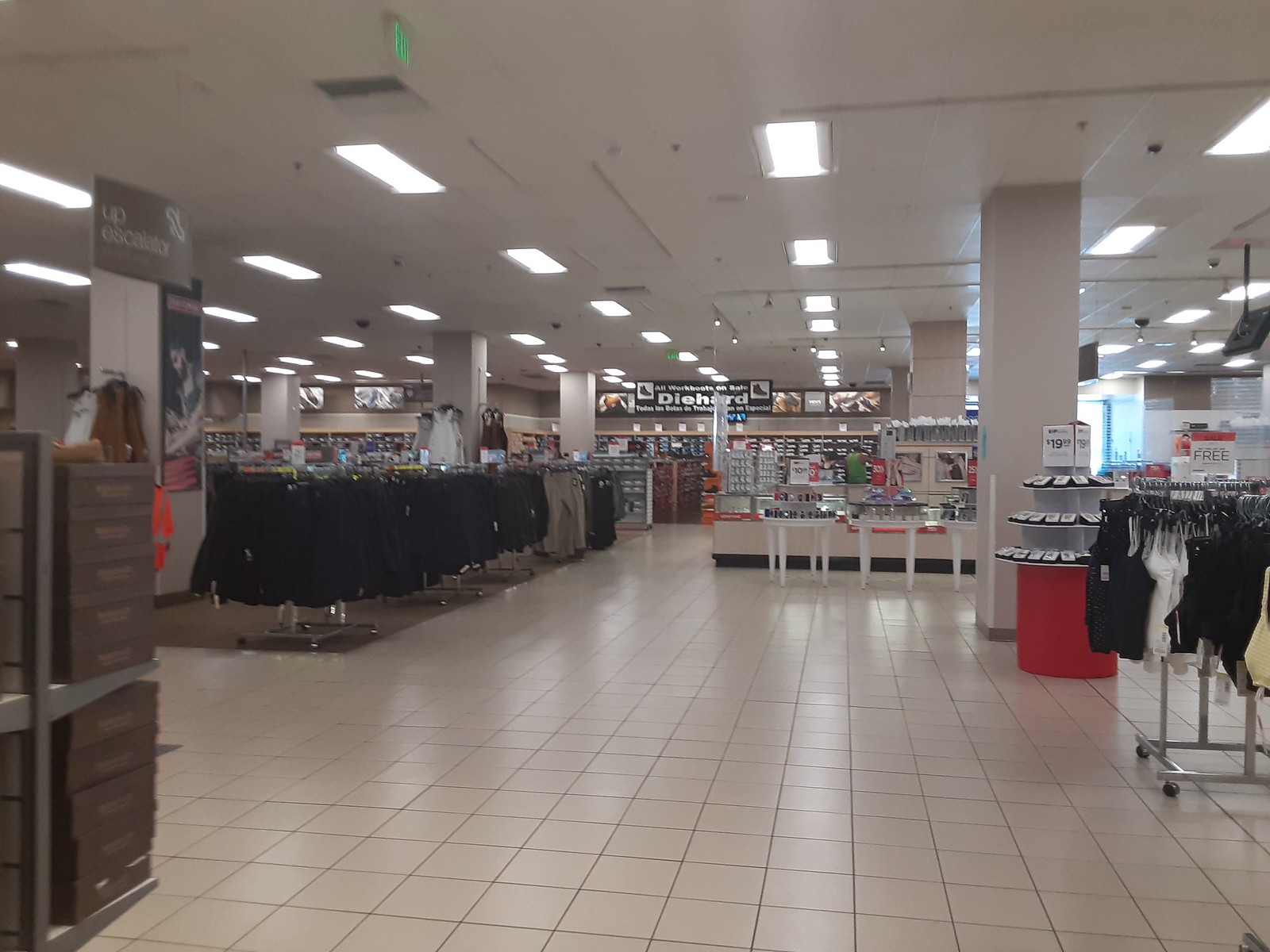A hauntingly empty clothing store within a mall features rows upon rows of meticulously arranged garments. In the center, a kiosk displays an assortment of jewelry, gleaming under the stark fluorescent lights. Towards the back of the store lies the shoe department, marked by a banner that reads "Clothing, Work Boots, Die Hard." This section includes a neatly organized wall of shoe boxes stored within cubbyholes. The entire store is illuminated by overhead fluorescent lights that cast a cold glow on the scene below. The floor is covered in white tile with dark grout lines adding contrast. 

In the foreground, a clothing rack brimming with black, white, and tan vests or camisoles — it's hard to tell — is topped with a prominent "FREE" sign, likely indicating a "Buy One, Get One Free" offer, although only the word "FREE" is visible. The eerie stillness is palpable, with no shoppers in sight.